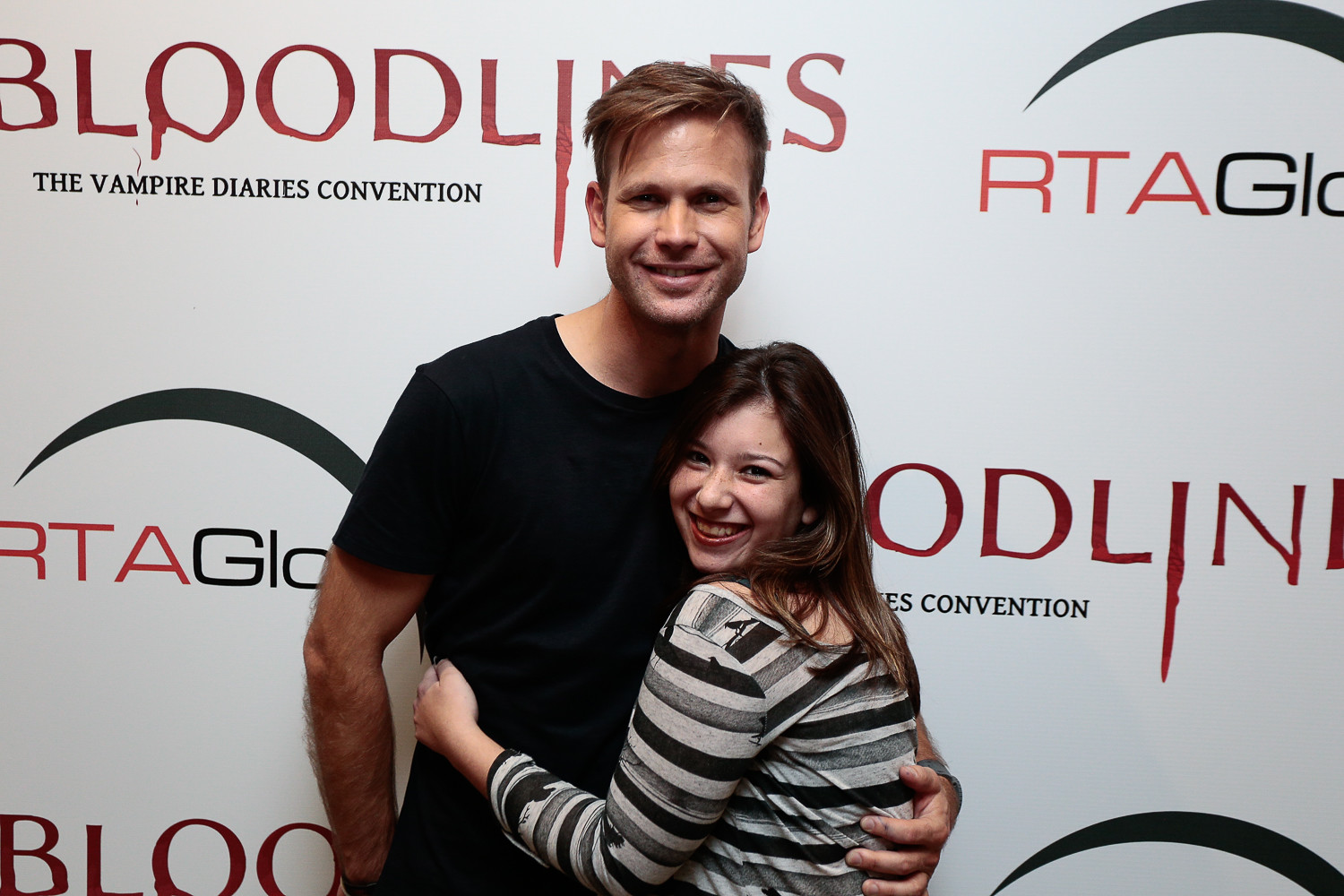In the photograph, a woman is warmly hugging a man, who appears to be a celebrity from the Vampire Diaries, during a meet and greet event. The backdrop is a white banner with the word "BLOODLINES" displayed prominently in red, blood-dripping capital letters, signifying the Vampire Diaries Convention. Directly beneath it, "The Vampire Diaries Convention" is written in black capital letters. The backdrop also includes the logo "RTA GLO" in alternating red and black colors.

The man, who is likely an actor from the show, is a Caucasian male with short blondish-brown hair, styled with a longer front part flopped to the side. He has some facial stubble and blonde arm hair. He is smiling and dressed in a plain black t-shirt. The woman he's hugging is noticeably shorter, with her head reaching his shoulder. She is a young Caucasian female, probably in her teens or early twenties, with long brown hair and wearing a black, white, and gray striped top. She is smiling widely, clearly thrilled to be in the moment.